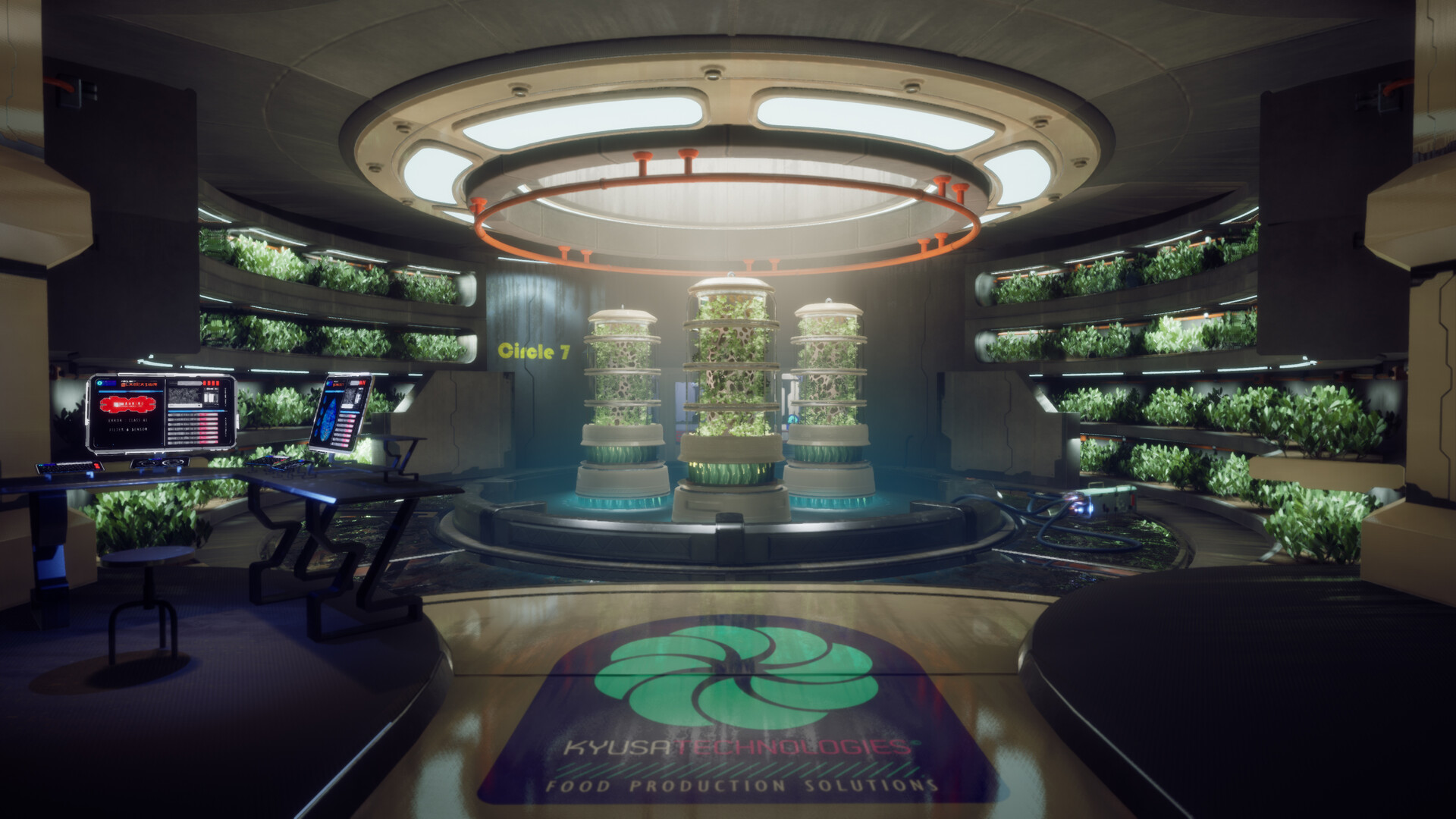The image is a 3D digital photograph showcasing a high-tech food production room, possibly from a company named CHI USA Technologies Food Production Solutions. The scene is set in a rectangular, horizontally aligned indoor space with a polished, tan-colored wooden floor. In the center of the room, three multi-tiered cylindrical columns host various plants, with each level separated by white plastic disks, and the base of each column is illuminated with a soft blue light. Surrounding these columns are curved shelves on the walls, also lined with well-lit plants under grow lights.

To the left-hand side of the image, a modern desk is accompanied by a small three-legged stool and features two futuristic computer monitors. The desks form an almost right-angle, facilitating easy access to both screens for a hypothetical user. Above the columns, a large circular lamp, supported by segmented rods, illuminates the plants below.

On the floor, centrally placed, is a logo depicting a stylized nautilus shape with crescent arcs nested within one another, and text reading "CHI USA Technologies Food Production Solutions." The background and overall room ambiance suggest a modern design with possible Asian influences, evidenced by the sleek, minimalist aesthetic and the curvature of the structures. Panels and geometrical shapes in varying shades of gray and tan add to this contemporary feel. The lighting in the room primarily highlights the plants, giving the entire scene a focused, almost laboratory-like atmosphere ideal for advanced agricultural research.